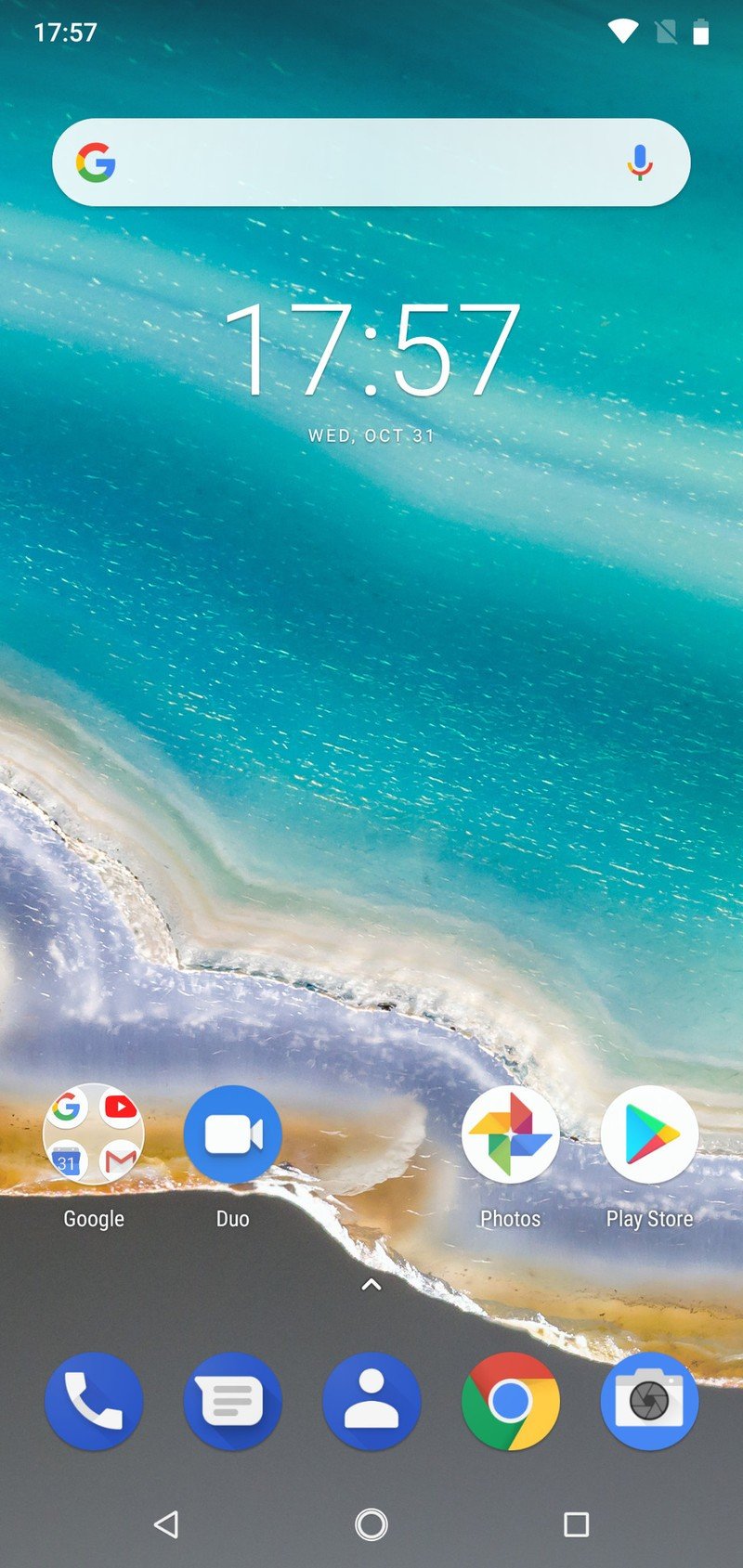The screenshot depicts the home screen of an Android phone. At the very top left corner, the time is displayed as 17:57 (5:57 PM). On the right side of the status bar, various icons are visible, including the WiFi symbol, a grayed-out file icon, and the battery indicator. Below the status bar is an empty Google search bar. Centrally located beneath the search bar, the time is shown again, with the date "Wednesday, October 31" displayed directly below it. The wallpaper is an aerial view of a beach, providing a scenic backdrop. Several app icons are visible on the home screen, predominantly consisting of Google applications.